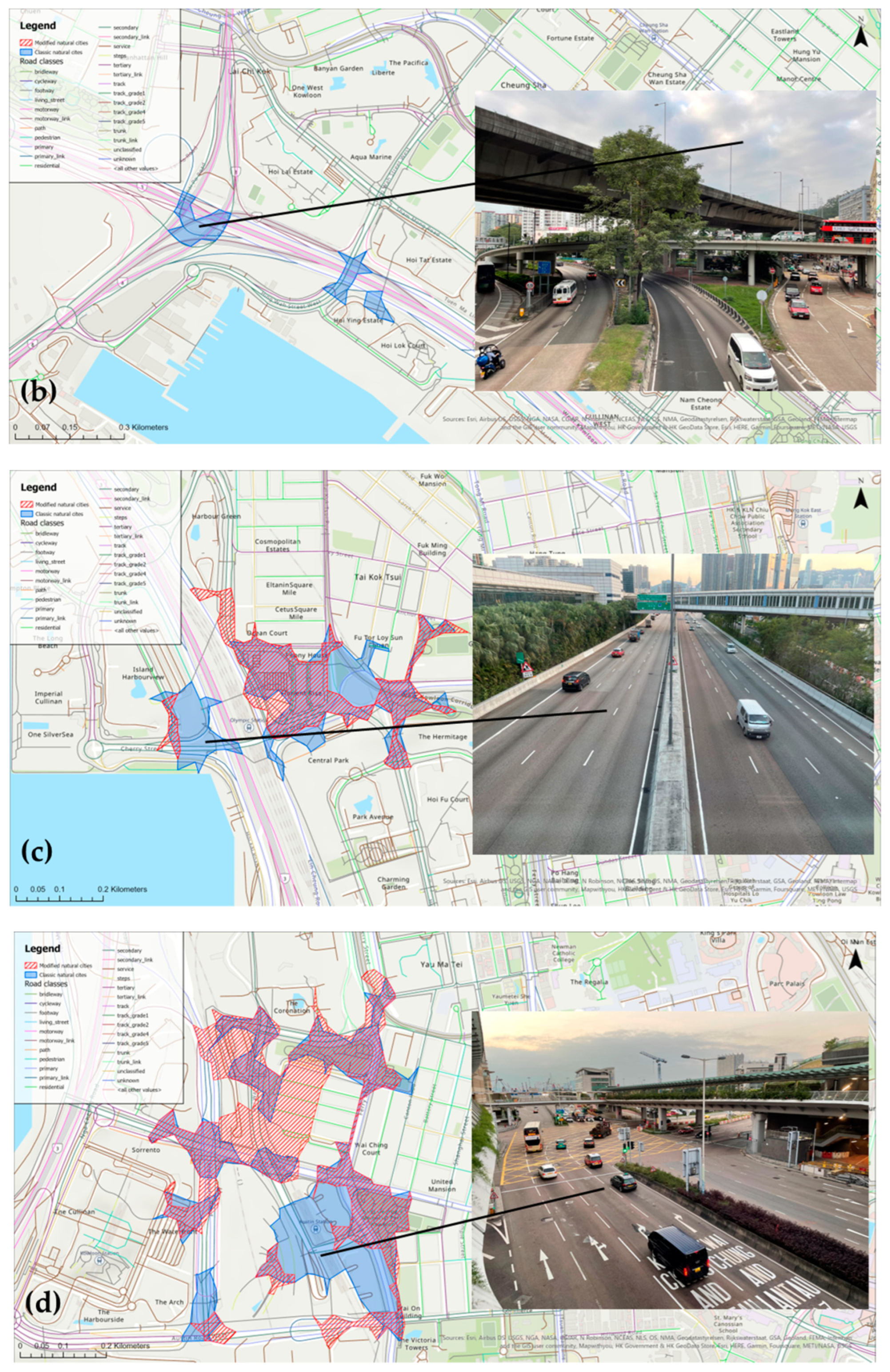This image presents three detailed maps identified as B, C, and D, each labeled in the lower left corner. The maps depict an urban harbor area with major highways but lack specifics on geographical location. Each map section contains an inset photograph to the right, illustrating specific segments of the highways shown: 

- Map B features an on-ramp to a freeway beneath two overpasses, populated with cars and buses, including a white minivan merging onto a four-lane freeway.
- Map C depicts a relatively empty stretch of an interstate highway with four lanes in each direction; a line connects the photograph to a specific point on the map.
- Map D shows a merging area where two four-lane highways converge, again with a line indicating the photograph's exact location on the map.

All maps include a legend in the upper left corner, detailing route information in pink and blue colors. Despite these details, the small text in the legend and the lack of an overarching label for the area make it difficult to identify the precise locations without prior familiarity.